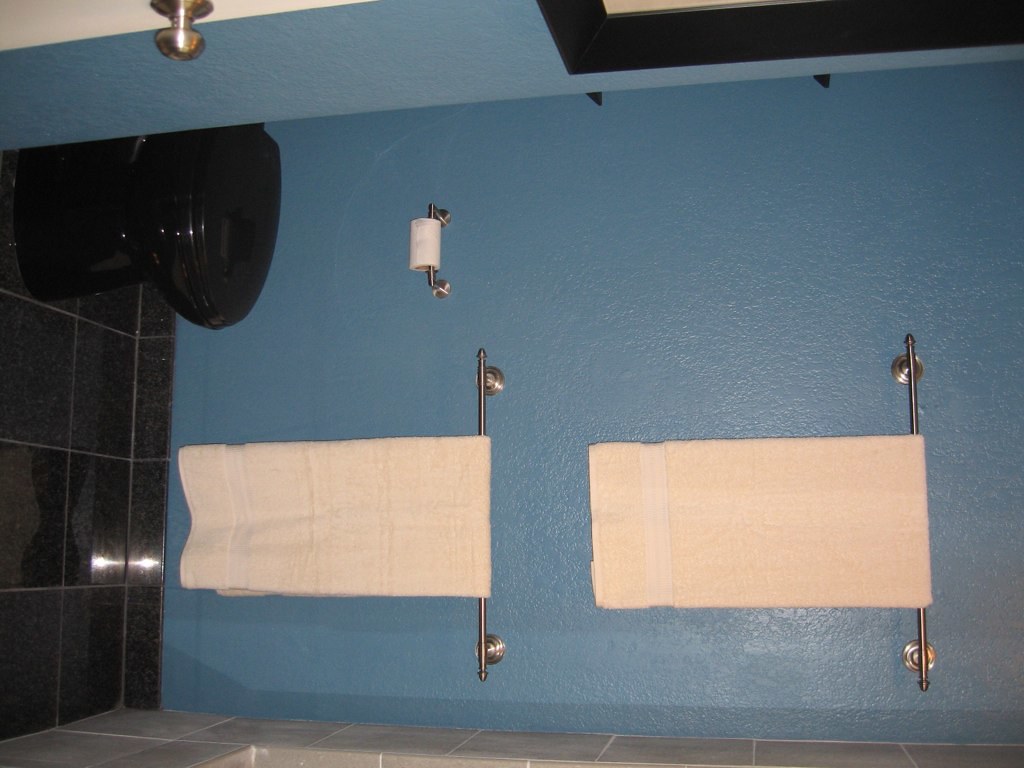The image is a sideways photograph of a bathroom, flipped 90 degrees to the right, making the left edge of the image appear as the bottom. The bathroom features a shiny blue wall that some might find unattractive. On what is now the top edge, there is a partially open white door with a stainless steel handle, revealing a sliver of the doorway. To the left of the door handle, there is a black-framed picture hanging on the wall. 

The main focus of the photograph is a black toilet with a closed lid, set against a backdrop of black tile flooring. Adjacent to the toilet is a toilet paper holder with a nearly depleted roll, mounted on a stainless steel bar. Above and to the right of the toilet are two horizontally-aligned towel racks made of stainless steel, each holding an off-white towel. These racks are positioned approximately three feet and six feet high, respectively. Additionally, the image hints at the presence of a bathtub and shower setup, characterized by gray-tiled walls.